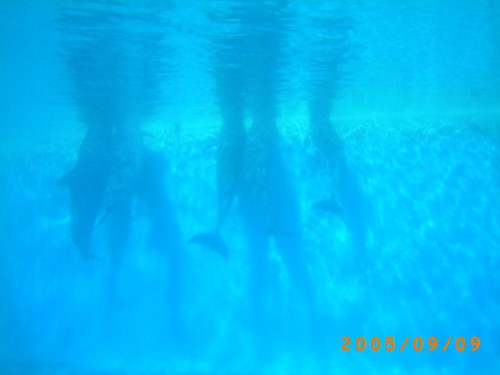This color photograph, taken underwater on September 9, 2005 (as indicated by the orange timestamp in the lower right corner), features a vibrant, bright turquoise blue scene. The surface of the water, about a third of the way up the frame, reveals ripples and light rays emanating from the sun above, creating a striking ripple effect. The subjects below are somewhat unclear due to the fuzzy focus, but we can discern several upright shapes that could be swimmers and sea creatures. The swimmers' legs and torsos are visible, though their heads are not, suggesting they are partially submerged. Accompanying them are at least three aquatic animals, possibly large fish or small sharks, with fanning tail fins clearly visible. Additionally, some shapes may be the shadows of dolphins, with at least seven of them appearing to peer above the water's surface. The overall lighting is enriched by the sunlight filtering through, creating a dynamic and slightly surreal underwater tableau.